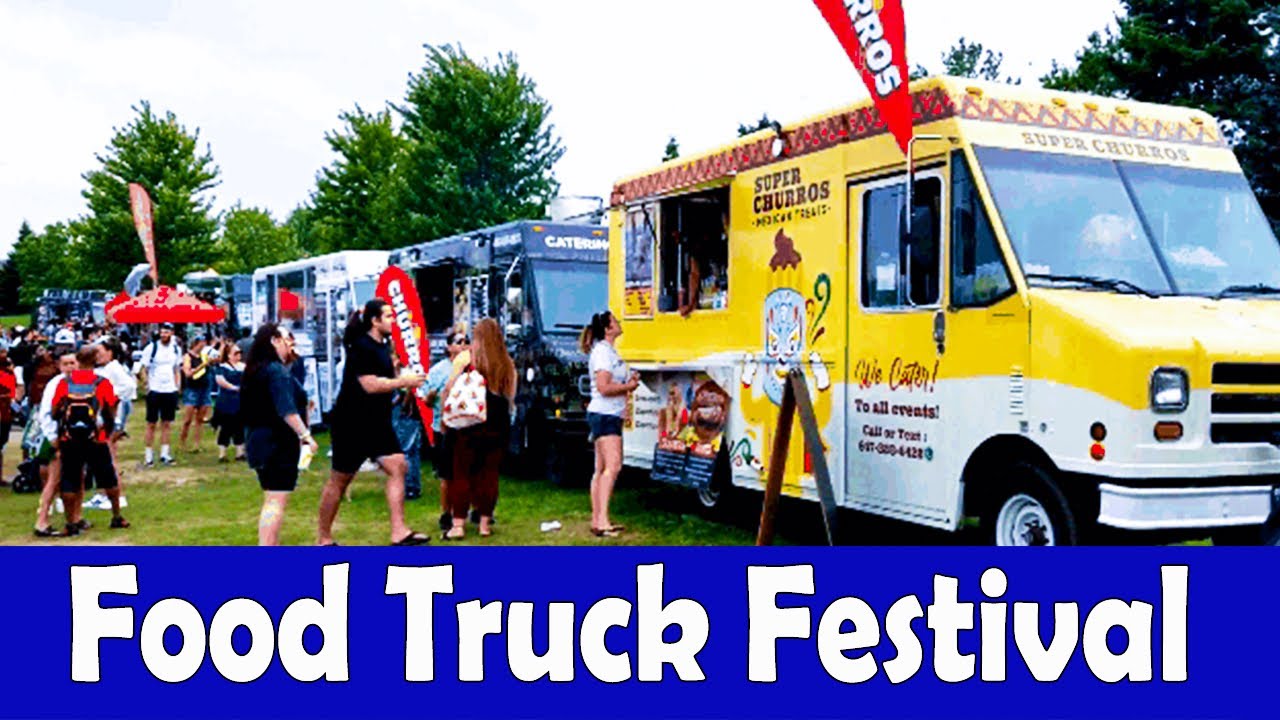The photograph captures a vibrant Food Truck Festival set in a grassy field beneath a canopy of leafy green trees, with a blown-out white sky overhead. A line of colorful food trucks stretches diagonally from the left side to the right, creating a lively and bustling atmosphere. The closest food truck is bright yellow with a white stripe at the bottom, prominently branded as "Super Churros" at both the top and front. Its door, adorned in red text, offers catering services with the message, "We cater to all events call or text 627-320-4422," accompanied by a whimsical figure of a churro-headed character wearing a blue mask and a chocolate cap. The subsequent food trucks vary in color, including black, white, and blue, diminishing in size as the line progresses into the distance. Enthusiastic attendees, clad in summery outfits including shorts and t-shirts, queue up at the windows, some carrying bags and backpacks. One individual stands out with a red umbrella. Below the image, a vivid blue rectangle spans the width, emblazoned with the event's name, "Food Truck Festival," in crisp white text, underscoring the festive scene above.